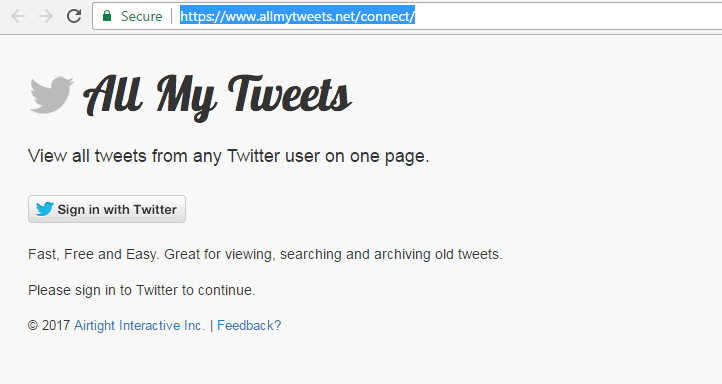This image depicts a partial web page, specifically from a computer screen. At the top, there is a search bar displaying the word "secure," followed by a highlighted URL beginning with "https://www.allmytweets.net/connect/," indicating a secure connection. Below the URL, the Twitter emblem featuring a gray bird facing right is prominently displayed, with its wings slightly uplifted.

The header of the page showcases the site name "All My Tweets" in elegant black lettering. Directly underneath, a tagline reads, "View all tweets from any Twitter user on one page," also in black font against a light-colored background.

A horizontal rectangle beneath the tagline houses another blue Twitter bird icon, signifying the option to "Sign in with Twitter." Below this sign-in invitation, the text "fast, free, and easy" is written in a gradient ranging from lighter black to dark gray. An additional informational line states, "Great for viewing, searching, and archiving old tweets. Please sign in to Twitter to continue."

The bottom of the image includes the site's copyright information in gray and blue letters, dated 2017. This overall design and information suggest an intuitive, user-friendly web service for managing Twitter content.